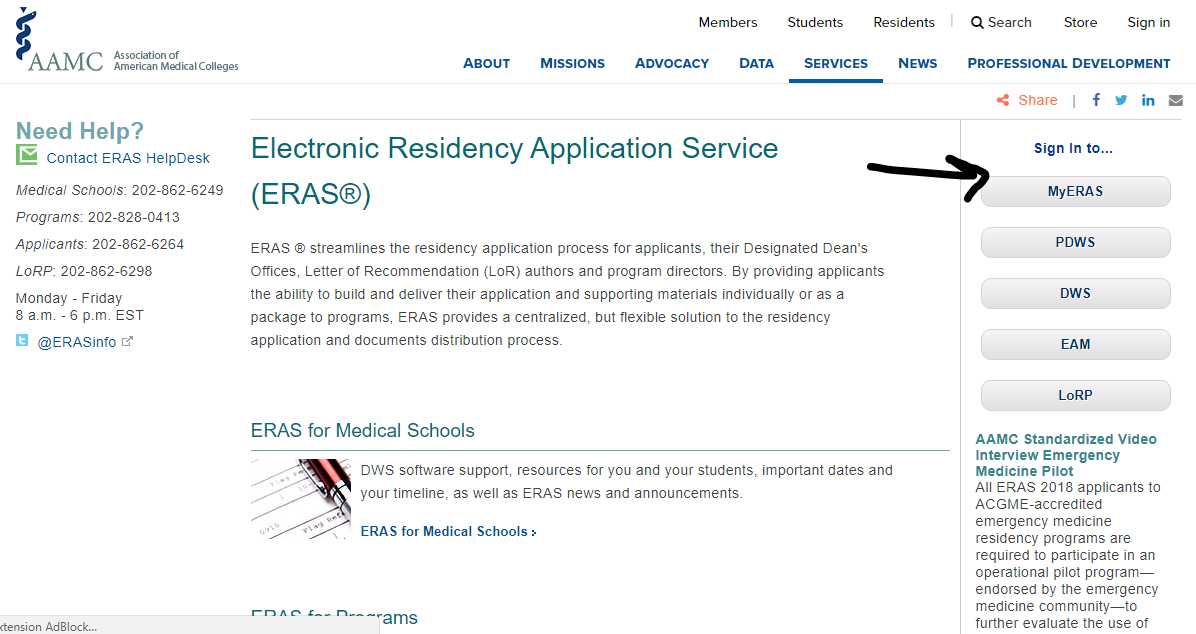Screenshot of the Association of American Medical Colleges (AAMC) Homepage

The screenshot captures the homepage of the Association of American Medical Colleges (AAMC) website. The overall design features a clean, white background with black or dark gray text and blue links, accented by a medium teal color used for header texts and other highlights.

At the very top right of the page, there is a navigation bar with the following links: "Members," "Students," "Residents," "Store," and "Sign In." A search bar is also located in this section for easy access to search functionality.

Just below the top navigation bar, a prominent menu is displayed, featuring larger, bold blue text for different categories, including "Missions," "Advocacy," "Data," "Services," "News," and "Professional Development."

On the left-hand side of the screen, there's a "Need Help?" section, providing various phone numbers and contact information, including their service hours which are from 8 AM to 5 PM Eastern Standard Time. There are four phone numbers listed, suggesting multiple points of contact. Additionally, their Twitter handle is mentioned as @ERASinfo.

In the central part of the screen, the key focus is on various articles and sections regarding the Electronic Residency Application Service (ERAS). One detailed segment explains how ERAS streamlines the residency application process for applicants, designated dean's office, letter of recommendation (LOR) authors, and program directors by offering the ability to build and deliver applications and support materials either individually or as packages to programs. ERAS is described as a centralized and flexible solution for managing the residency application and document distribution process.

A notable visual element is the black arrow drawn on the screen, pointing towards a link labeled "MyERAS." This link is situated beneath a header that reads "Sign into" on the right side of the screen. Below this header, other links include "MyERAS," "PDWS," "DWS," "EAM," and "LORP."